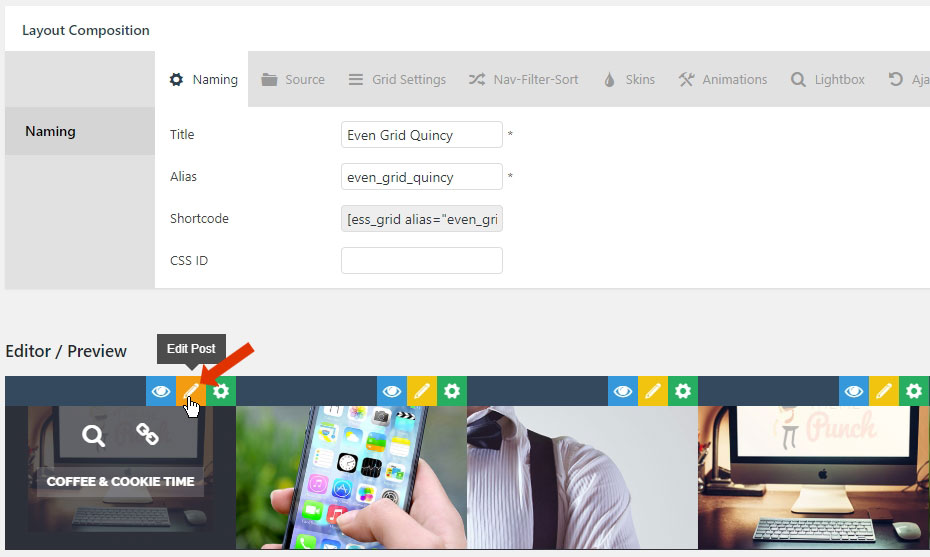In the image, we are presented with a detailed layout composition. The background transitions from white at the top to gray linings on the left and over the top portion, creating a structured frame. On the left side in black font, the phrase "Layout Composition" is prominently displayed.

The top section is filled with numerous labels in a hierarchical format, starting with "Naming," "Source," "Grid Settings," "Nav," "Filter," "Sort," "Skins," "Animations," and "Lightbox." Some text appears to be truncated and potentially incomplete. Under the "Naming" section, highlighted in white with a gray sidebar, the word "Title" is specified. Adjacent to this is a text box that contains "even grid Quincy," followed by another line labelled "Alias" which reads "even_grid_Quincy" in a similar box. Below this line, a shortcode is displayed: "[S_grid, alias=even_grid]". The "CSS ID" is shown next but remains empty.

At the bottom section of the layout, the words "Editor / Preview" are displayed. Next to it, a gray box with white font says "Edit Post." There is a red arrow pointing to an orange box with a white finger and pencil icon, symbolizing editing. Adjacent to it is a blue box with a white eye icon, possibly denoting a preview function, and a green box to the right featuring a search icon. This sequence of icons repeats itself three more times horizontally towards the right.

Below this composition, another visual segment shows a person holding a phone and touching the music button, recognizable by its red and white music note icon. To the left of this, white font reads "Coffee and Cookie Time," accompanied by a search icon and a chain link icon, all against a gray background with respective white and gray-square outlines. To the far right, there appears to be a close-up image of a man's shirt with black straps, likely part of a backpack or other accessory. Finally, on the rightmost side is an Apple computer monitor displaying the word "Pinch" in light brown text, set atop a brown wooden table with a gray wireless keypad and mouse, prominently featuring the Apple logo.

This detailed layout effectively conveys a complex arrangement of design elements, iconography, and interactive buttons within a structured framework.